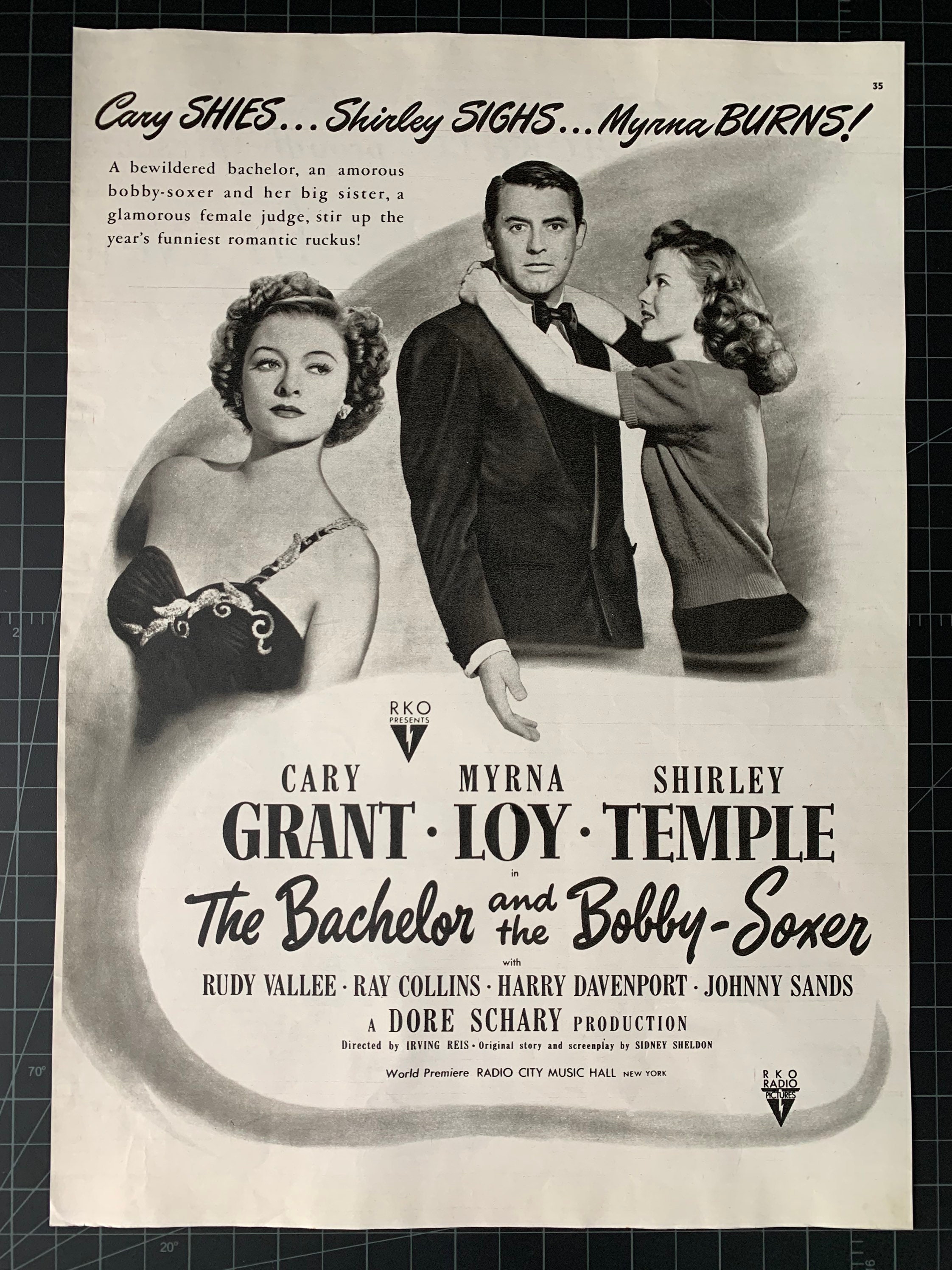This black and white poster for the 1947 film *The Bachelor and the Bobby Soxer* prominently features its three stars: Cary Grant, Myrna Loy, and a teenage Shirley Temple. At the top, playful text reads "Cary Shys, Shirley Size, Myrna Burns," setting a comedic tone. The poster's tagline below describes the plot: "A bewildered bachelor, an amorous Bobby Soxer, and her big sister, a glamorous female judge, stir up the year's funniest romantic ruckus." Visually, the poster showcases the three main actors: a woman on the left wearing a strapless black dress, a man in the center in a black suit with a bow tie, and another woman on the right in a short-sleeved sweater and dark bottoms. Additional cast members such as Rudy Vallee, Ray Collins, Harry Davenport, and Johnny Sands are listed alongside production credits for Dore Schary. Directed by Irving Reis, with an original story and screenplay by Sidney Sheldon, the film’s world premiere was held at Radio City Music Hall. The layout includes the names of the major players at the top, the film title in the center, and secondary details towards the bottom. The poster is affixed to a black board marked with white lines and measurements, suggesting an engineer's drafting surface.